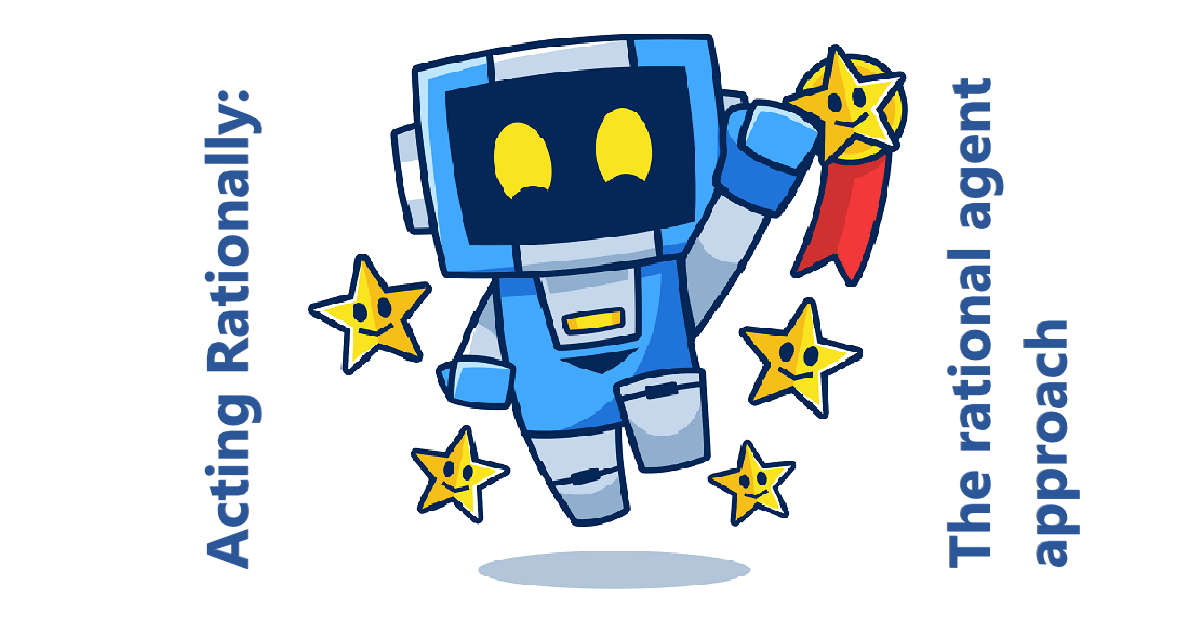A vibrant banner on a website features a positive and educational message. On the left side, the text reads "Acting Rationally," while on the right, it says "The Rational Agent Approach." Centrally located, a cartoon-style robot is depicted in a dynamic, celebratory pose, as if running and jumping with one hand raised in triumph. Surrounding the robot are several smiling stars, symbolizing awards or recognition. Notably, the star in the upper right corner is adorned with a gold coin and a red ribbon hanging below it, enhancing its award-like appearance. This cheerful and informative banner aims to teach the importance of rational decision-making and thought processes, encouraging viewers to act rationally and think things through rather than jumping to conclusions.